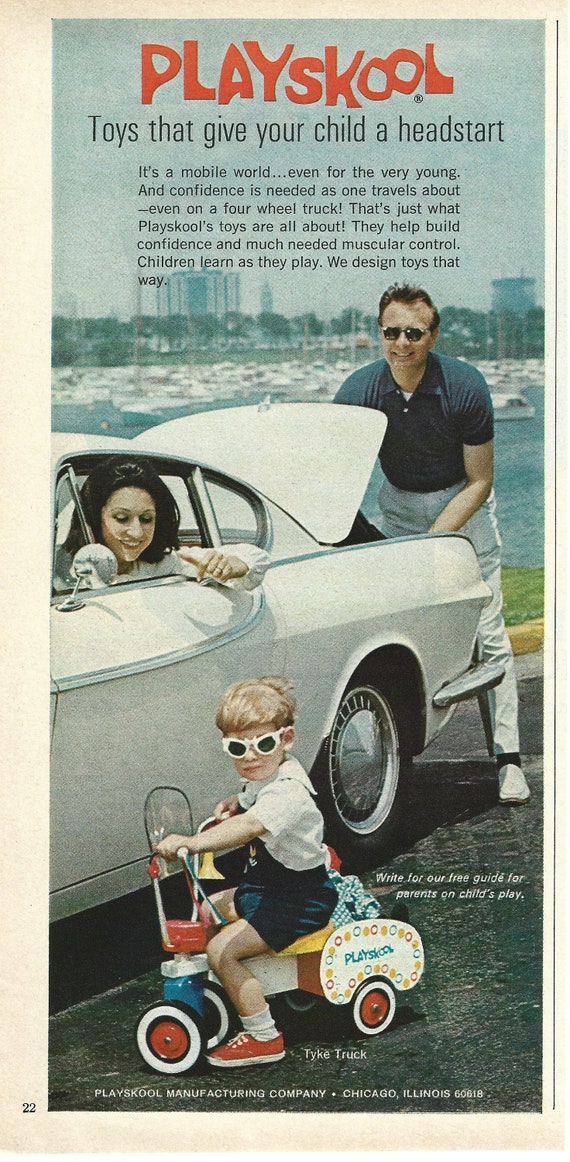The image showcases a vintage PlaySchool advertisement prominently featuring the PlaySchool logo in red, accompanied by the slogan "Toys That Give Your Child a Head Start". The scene is set near a waterfront with boats and numerous buildings in the background. In the foreground, a playful family moment is depicted: a man with short brown hair, wearing sunglasses, a navy blue collared shirt, white pants, and white shoes, is seen smiling while rummaging through the trunk of a white car. Inside the car, a woman with long black hair donning a long-sleeved white shirt is pointing and looking affectionately at her child. The child, with shaggy blonde hair, blue overalls, a white short-sleeved shirt, and white glasses, is joyfully riding a colorful PlaySchool toy truck. The toy truck features red wheels, a yellow seat, chrome handlebars, and the PlaySchool branding on its side. The text on the ad emphasizes the role of PlaySchool toys in fostering confidence and essential motor skills in children. It reads, "It's a mobile world, even for the very young. Confidence is needed as one travels about, even on a four-wheeled truck. That's just what PlaySchool toys are all about – they help build confidence and much-needed muscular control. Children learn as they play. We design the toys that way."